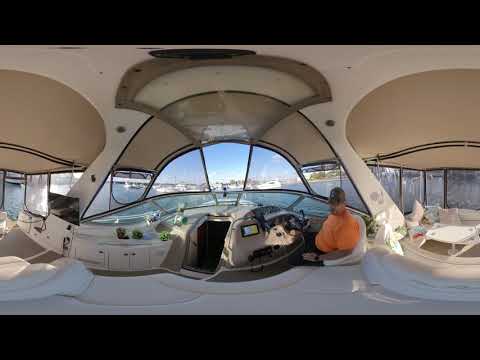The image is a 360-degree view of the inside of a luxurious yacht, exuding an atmosphere of elegance and comfort. At the center of the scene, there is a man in a bright orange shirt, sporting a dark baseball cap and a watch, sitting in a white cushioned chair. The interior features predominantly white decor with some tan accents on the ceiling, enhancing its posh and clean appearance. Surrounding the space are large windows at both the front and back, offering expansive views of the harbor with other boats visible. The man appears relaxed, seated near the yacht's control area, turned slightly to the left in an open seating stance. To his right, there is a cozy seating area with cushioned seats, perfect for relaxation. The outside view showcases a beautiful teal blue ocean and a light blue sky, indicating a pleasant day on the water.